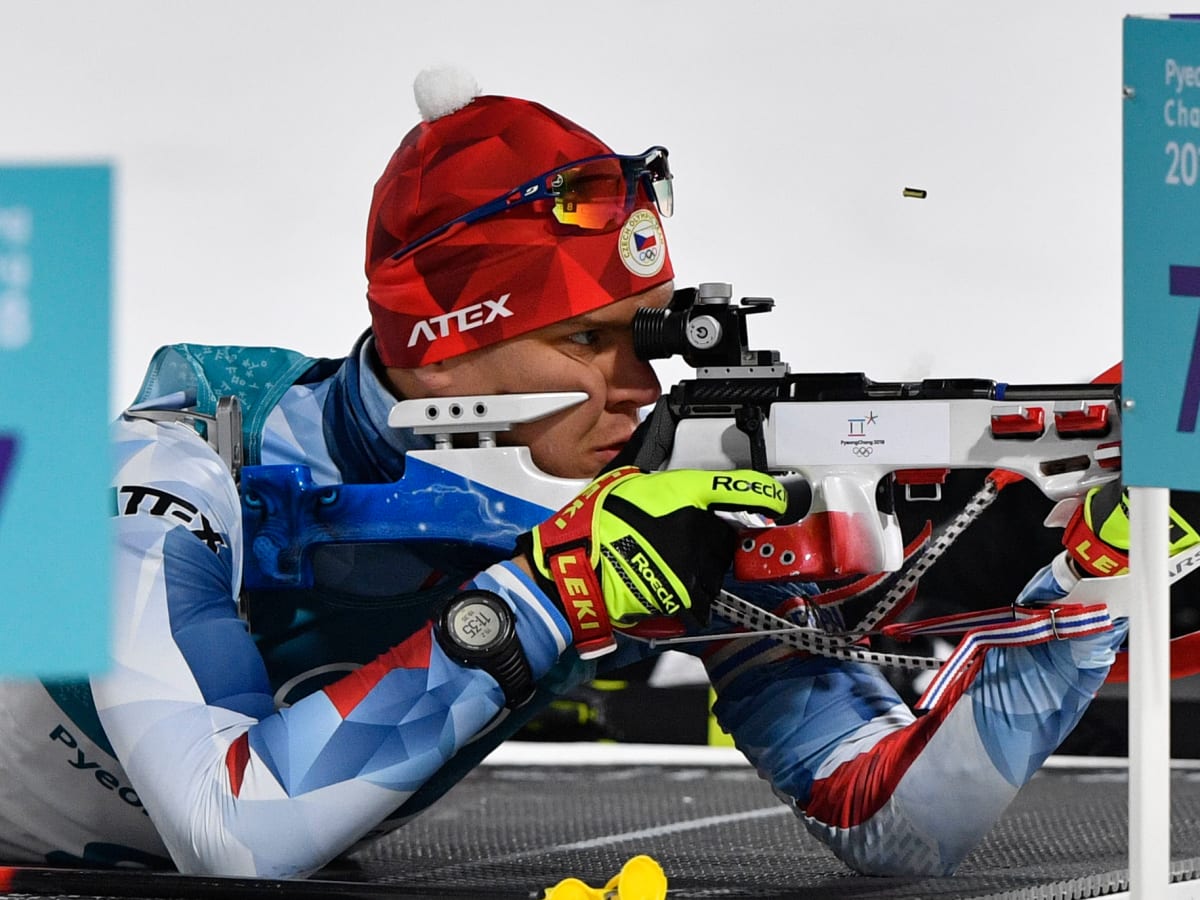This color photograph captures a sports shooter, a white male, in action during what appears to be an Olympic-type event. He is crouching, with his elbows resting on a black, mesh-like surface with white lines, intently aiming a white rifle accented with blue paint at the back and a black scope. The shooter is dressed in a tight-fitting athletic suit that is blue, white, red, and black, displaying some unreadable text. He wears a distinctive red sports beanie featuring the word "A-TEX" in white and a small white pom-pom. A pair of sports sunglasses rests on his forehead, just above the beanie. His gloves are neon yellow with red straps, emblazoned with the words "Rokey" and "Leckie" in black text. A black digital watch showing the time 11:35 adorns his right wrist. Behind him, there is a white wall and a partially visible blue sign with some unreadable white and blue text.